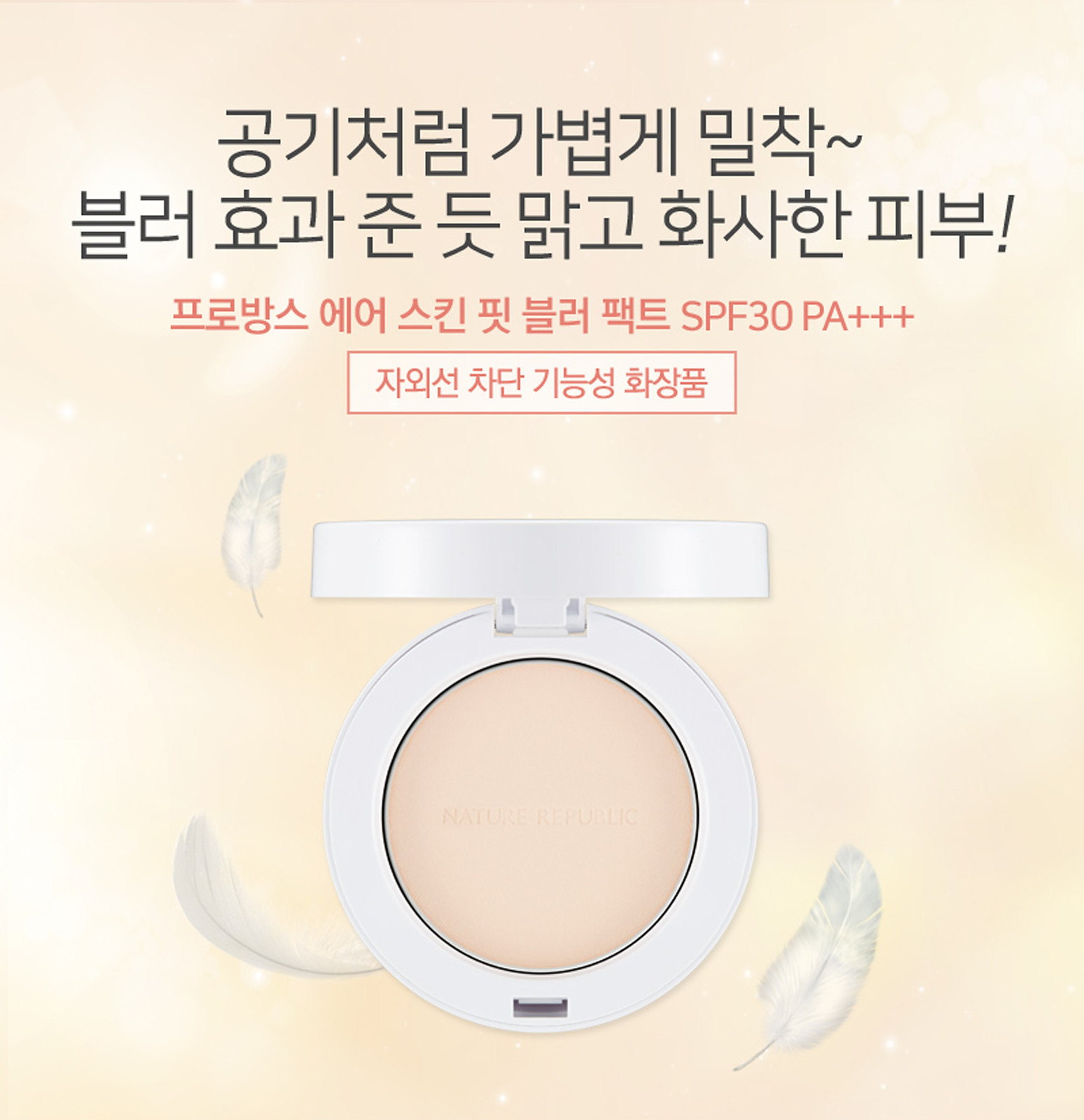The advertising poster for Facial Foundation Makeup Powder features a light yellowish, cream-colored background adorned with small white spots. At the very top, there are three rows of text written in Korean. The first two rows of Korean characters are in bold black font and at the end has an exclamation point. Below these, there is a third row of smaller, red Korean text, followed by another line of even smaller red text, which is encapsulated within a white rectangle outlined in red. Additionally, the poster mentions that the product boasts SPF 30 PA++, indicating its sun protection factor.

The main focal point of the advertisement is a compact of powder foundation, which is light beige, suitable for a pale complexion, and housed in a white case. This compact is open, allowing a view of the foundation inside. Elegantly complementing the scene, three delicate white feathers—varying in size from small to medium to large—are gracefully scattered around the compact. These feathers appear greyish-white and add a touch of softness and beauty to the presentation of the makeup product.